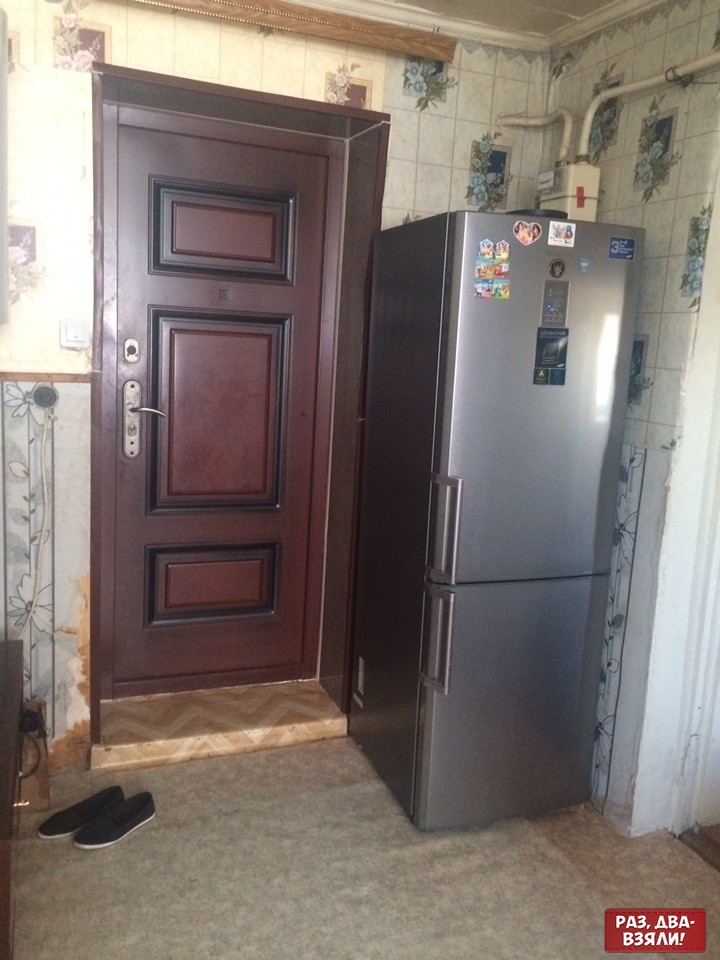This photograph captures a corner of a kitchen, prominently featuring a dark gray stainless steel refrigerator with silver handles, where the larger upper compartment is the fridge and the smaller lower compartment is the freezer. The refrigerator's front is adorned with various magnets, a photograph, and a notable blue rectangle with a silver "3" in the upper right corner. Positioned to the left of the refrigerator is a robust, dark reddish-brown wooden door with a long gold-plated handle and deadbolt, framed by a chocolate brown door frame. The kitchen walls present a mix of gray tile and floral-patterned wallpaper in cream, tan, and red hues. On the floor, a pair of black shoes with white soles is noticeable beneath the door, contrasting the brown carpet. The intricate details in this scene, from the decorative elements on the refrigerator to the texture and colors of the surrounding structures, evoke a homely yet cluttered ambiance.